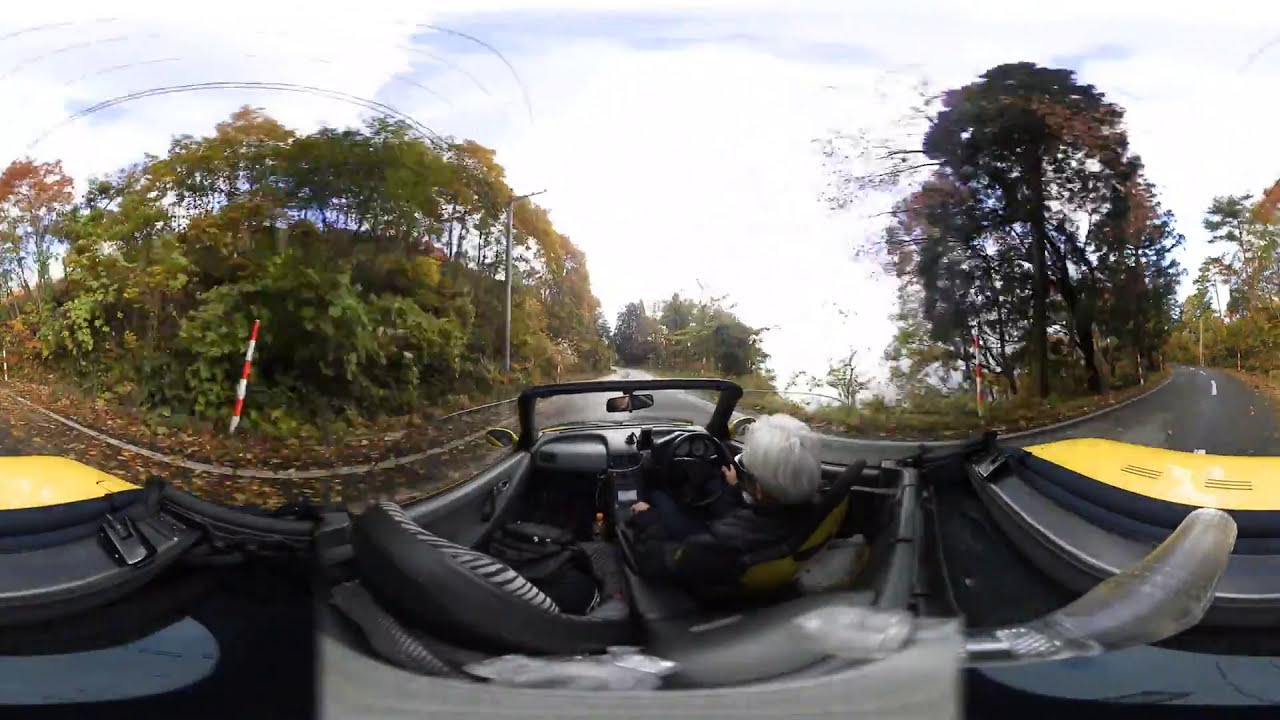In this dynamic panoramic photograph, a person is seen driving a yellow sports convertible with the top down along a tree-lined, two-lane road. The individual, who has long gray hair and is dressed in a black jacket and sunglasses, is seated on the right-hand side of the car, suggesting the location might be in Great Britain or another European country where vehicles drive on the left. The convertible’s windshield is accented with black, matching its interior. The car is navigating a slight curve in the road, emphasized by the panoramic and fisheye lens effect that blurs the road’s continuation to both sides, almost like a double exposure.

The day appears overcast, with a white sky dotted by large, puffy clouds and hints of blue peeking through. The road is bordered by dense groves of trees, adding to the serene countryside atmosphere. An orange and white pole stands by a guardrail on the left side of the road, punctuating the fully tree-lined scenery. The camera is mounted from the back seat, giving a clear view of the sole driver, and highlighting the empty passenger seat except for a bag on the driver's left. Despite the overcast sky, there are shadows on the trees, indicating the presence of diffuse sunlight. There are no other vehicles visible, suggesting a peaceful, solitary ride through the picturesque landscape.